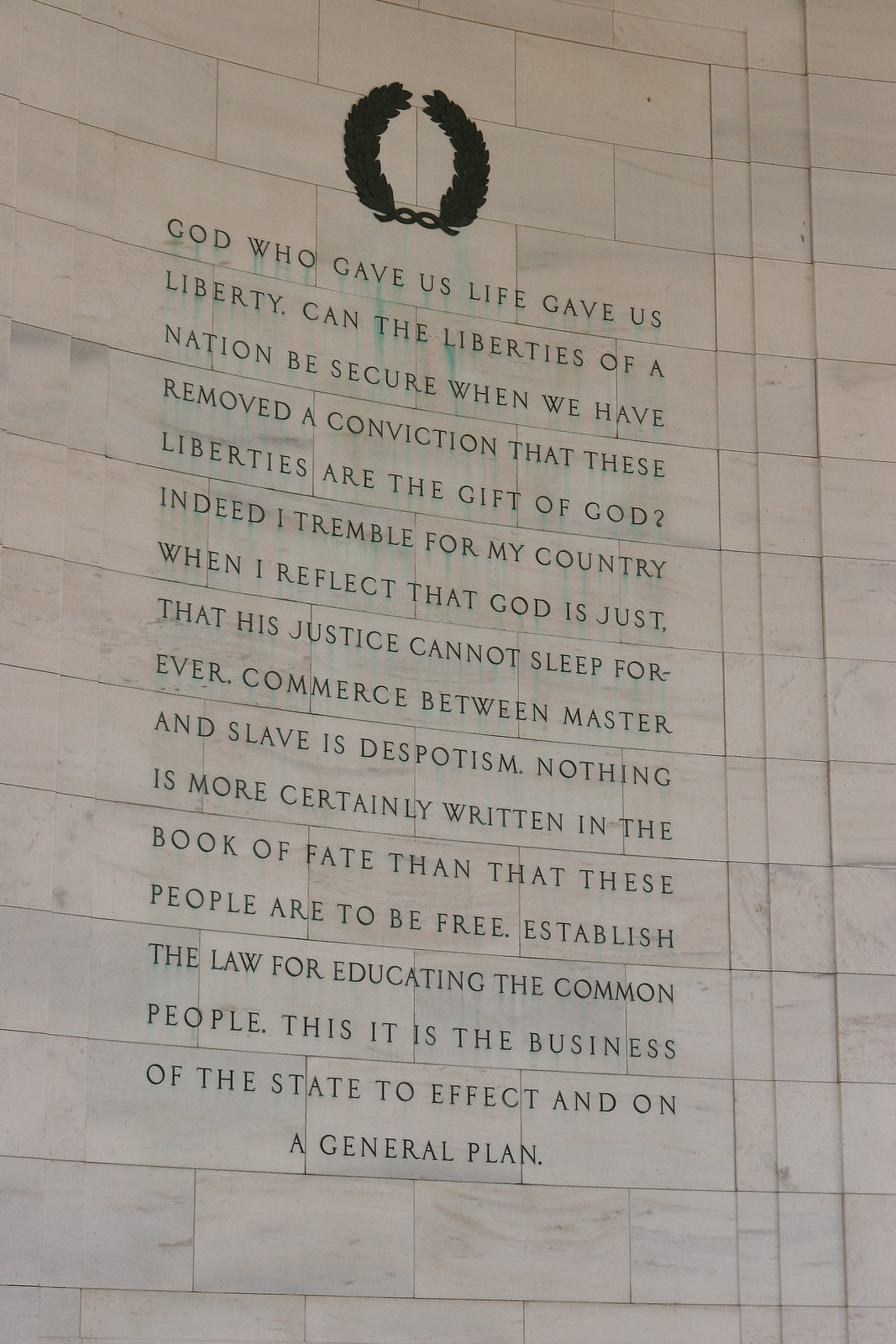The image depicts a large marble wall, composed of light-colored stones arranged in a brick pattern, which occupies the entire background. Prominently displayed at the top of the wall is a black silhouette of a wreath. Centered beneath the wreath is a poignant black text inscription. The text reads: "God who gave us life gave us liberty. Can the liberties of a nation be secure when we have removed a conviction that these liberties are the gift of God? Indeed, I tremble for my country when I reflect that God is just, that his justice cannot sleep forever. Commerce between master and slave is despotism. Nothing is more certainly written in the book of fate than that these people are to be free. Establish the law for educating the common people. This it is the business of the state to effect, and on a general plan." The wall appears to be part of a governmental building, potentially offering an atmosphere of solemn reflection on the principles of liberty and justice.